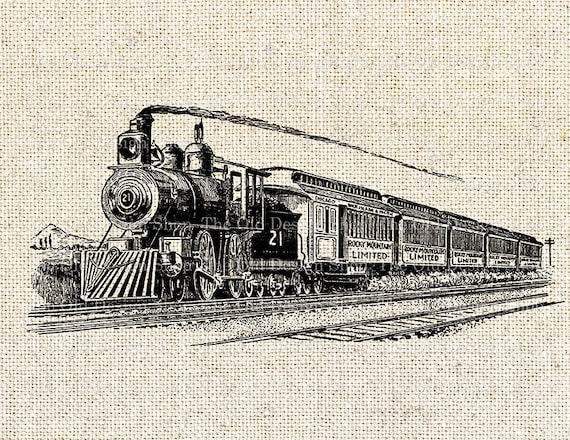This is a detailed black and white image of an old-fashioned locomotive, appearing to be an embossed ink drawing on a burlap or tan canvas material. The locomotive, marked with the number 21 on its rounded front engine, is producing a long line of steam from its smokestack trailing back toward the train cars. The train, labeled "Rocky Mountain Limited" on each of its five cars, travels on tracks with a parallel, empty set of tracks beside it. Distinguishable elements of the train include a prominent cow catcher at the front. The background suggests a western landscape with visible cacti, possibly a mesa or hill, and patches of sagebrush near the tracks, enhancing the rustic and historical feel of the scene.